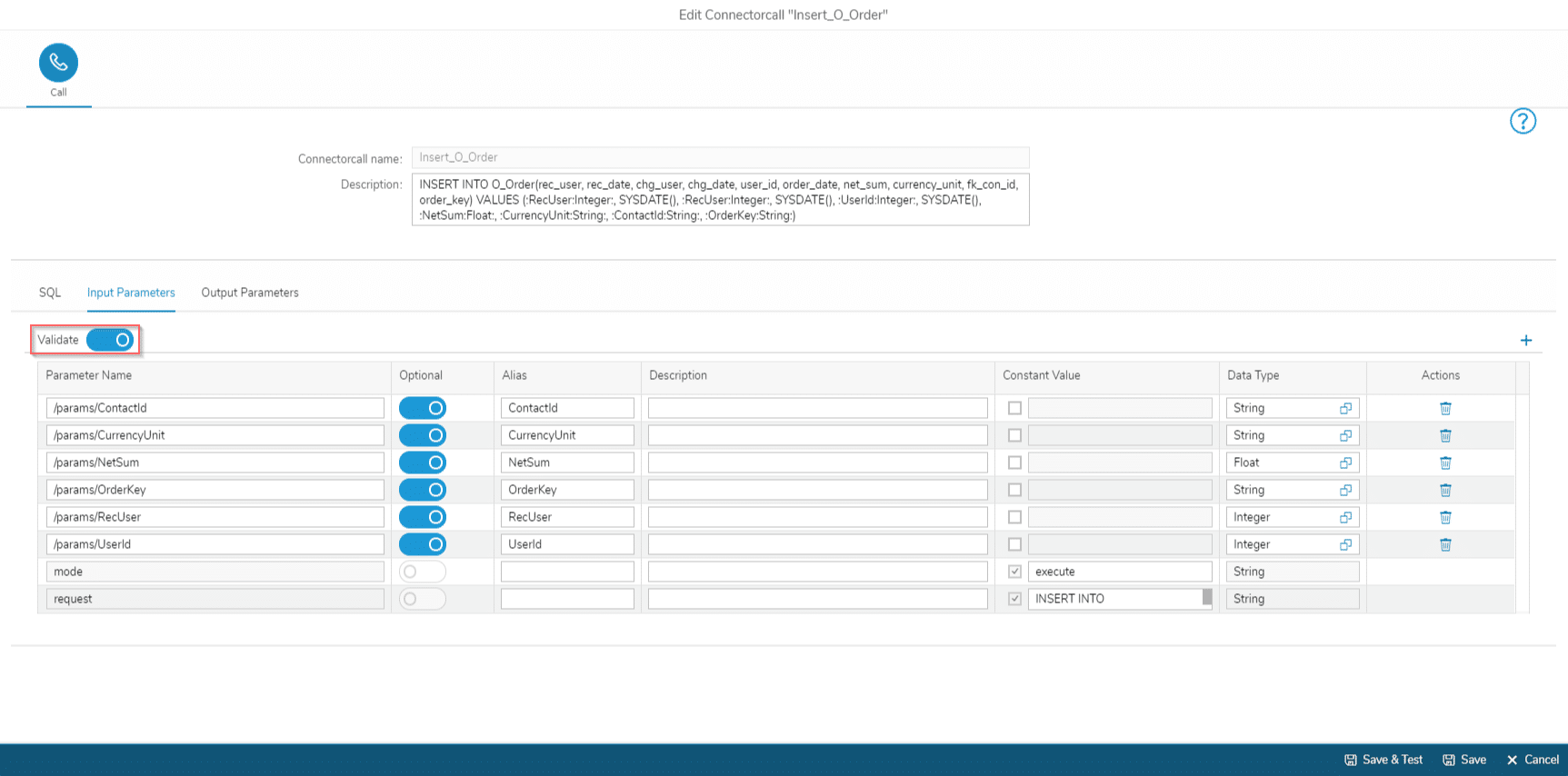The image is a screenshot of an application interface featuring a primarily white background. Centrally positioned at the top of the image, the text reads "Edit Connect or Call," formatted much like a single phrase. Directly below this header, aligned to the left side, is a blue circular icon with a white phone symbol inside it. Beneath this icon, the label "Call" is displayed.

Further down the interface, a highlighted section is visible. Within this section, under the heading "Input Parameters," a tickable toggle switch labeled "Validate" is prominently featured. This toggle switch is currently activated, indicated by its blue color; when deactivated, it turns white. Following the "Validate" toggle, a list of various parameters is presented, with most of their respective toggle switches also turned on, displaying the blue color.

Between the "Call" icon at the top and the list of parameters below, there is a box containing a string of code. This box is situated between the toggle switches and the "Call" button or icon mentioned earlier, serving as a separator and likely containing relevant code for the application's functionality.